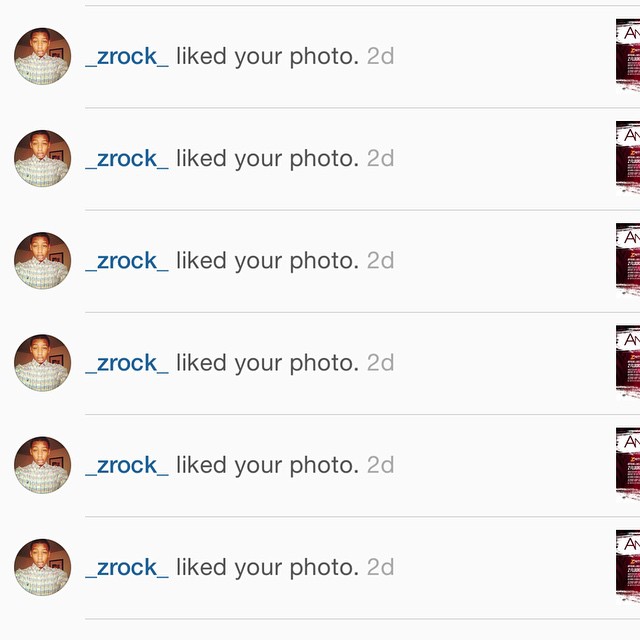The screenshot captures a series of interactions from Instagram, showing user Zrock repeatedly liking photos. There are six identical notifications, each stating "Zrock liked your photo" followed by "2 days ago." Zrock's profile picture, which is visible in each notification, features an African American man wearing a plaid collared shirt, looking directly at the camera. The username "Zrock" is highlighted in blue, and the rest of the text is in black. The image includes a partially visible letter "A" on the far right of each notification line, though its context is unclear.